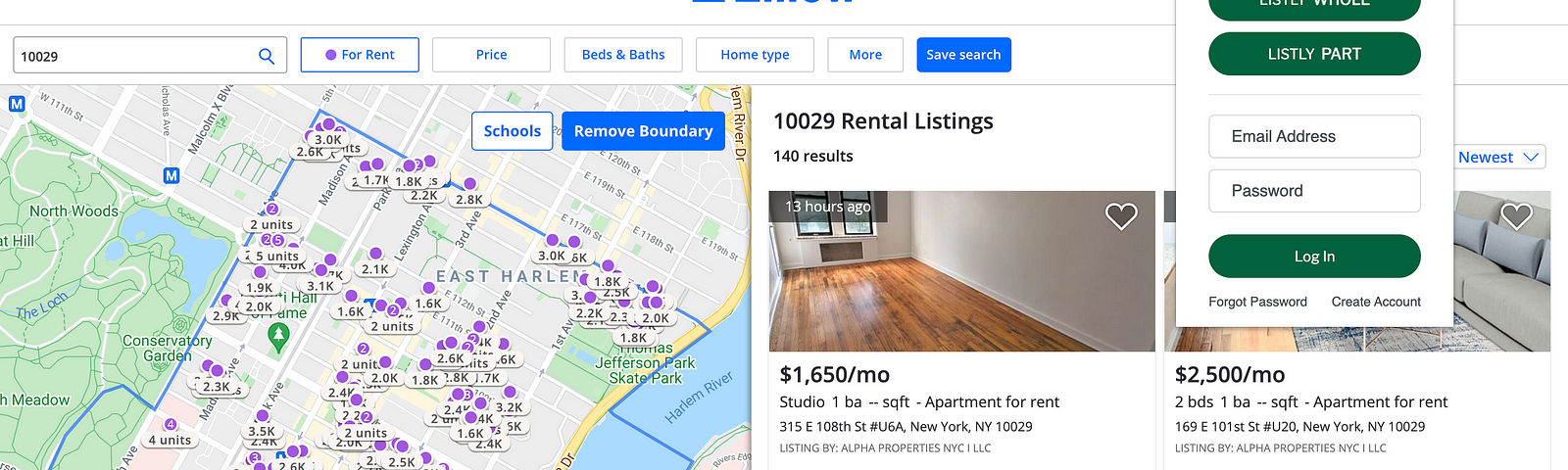This image appears to be a cropped screenshot from a real estate website, possibly showcasing rental listings. The image itself is elongated, approximately three to four times longer than it is tall. At the top of the screenshot, there is a white header featuring a search box with a black border, located in the top left corner. The search box seems to include a zip code, likely 10019, although it is not entirely clear. Adjacent to the search box, there is a blue-bordered button labeled "For Rent" highlighted in blue, surrounded by purple dots. Additional filters like "Price," "Beds and Baths," "Home Type," and "More" are displayed with black borders and blue font, indicating they are unselected.

Beneath these filters, the main section of the screenshot displays search results, presumably focusing on East Harlem. The area is dotted with numerous purple markers representing property prices. To the right of the map, there is a listing summary that reads "10029 rental listings" with a count of 140 results. Featured prominently is a photograph of an interior space, showcasing sleek dark gray or dark brown wooden floors and gray walls, with a rental price of $1,650 per month. Another partial listing, priced at $2,500 per month, offers a glimpse of a couch, though it is partially obscured by the search menu.